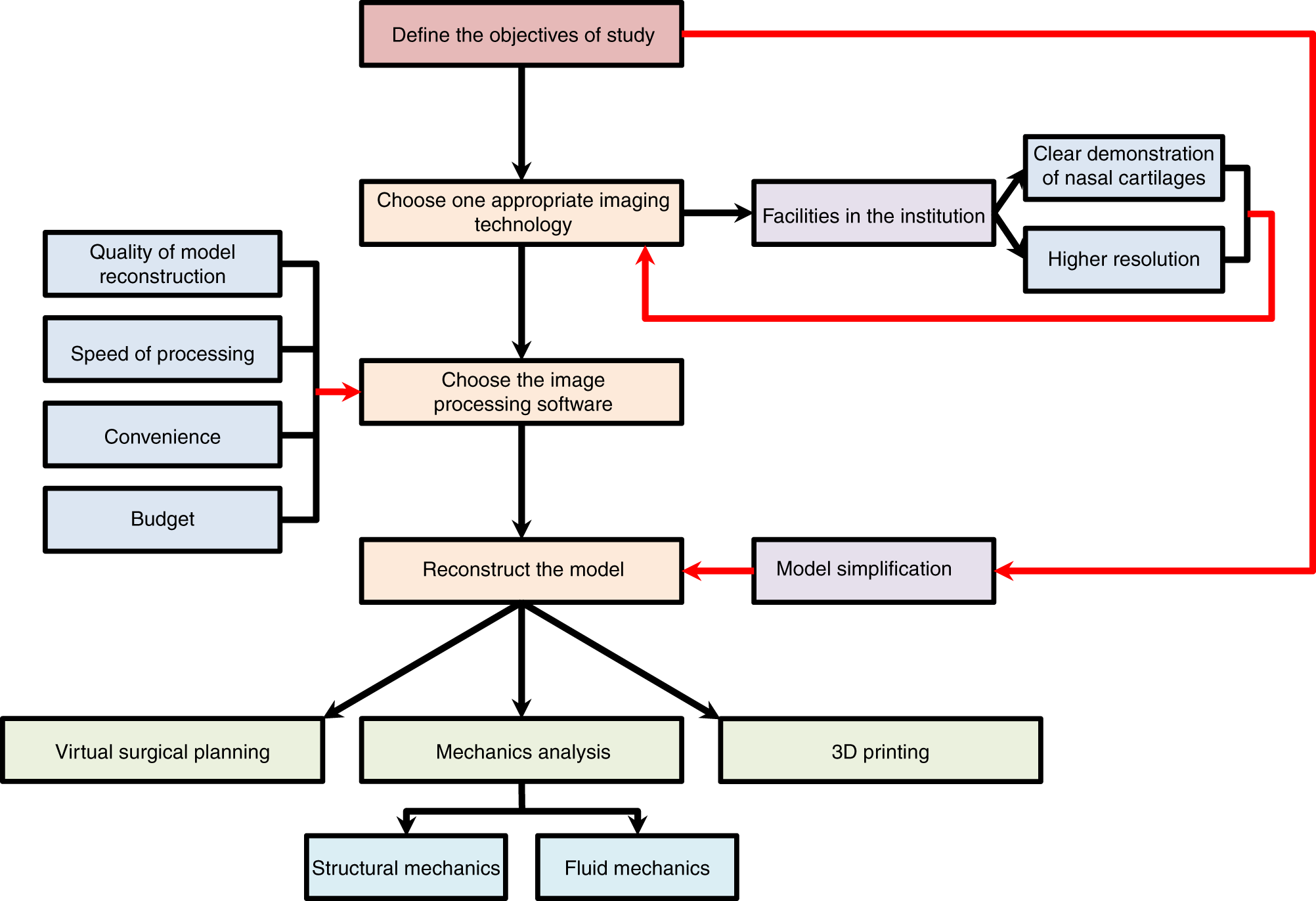This detailed flowchart illustrates the step-by-step process of conducting a study, starting with defining the objectives in a pink box. Following this, you choose one appropriate imaging technology, as indicated by a connected arrow leading to a peach box. Next, the selection of image processing software is the focus, followed by the reconstruction of the model, both denoted by additional peach boxes. From here, the process branches into three sage-colored boxes, offering paths for virtual surgical planning, mechanics analysis, and 3D printing. Mechanics analysis further splits into two blue boxes, detailing structural mechanics and fluid mechanics.

Alternative flows provide additional context to the central column. A red arrow from the initial step, defining the objectives, diverts to the model simplification box, which eventually reconnects to the reconstruct the model step. From choose one appropriate imaging technology, a rightward arrow points to a purple box labeled facilities in the institution, which splits into two subordinate boxes highlighting clear demonstration of nasal cartilages and higher resolution, both reconnecting to the imaging technology step.

Additionally, on the left side, there's a secondary vertical column of blue boxes outlining factors such as quality of model reconstruction, speed of processing, convenience, and budget, which all circle back to the choice of image processing software. This intricate diagram with multi-colored boxes and arrows provides a comprehensive view of the decision-making process required for study planning and execution, highlighted by the interactions between various factors that influence each step.